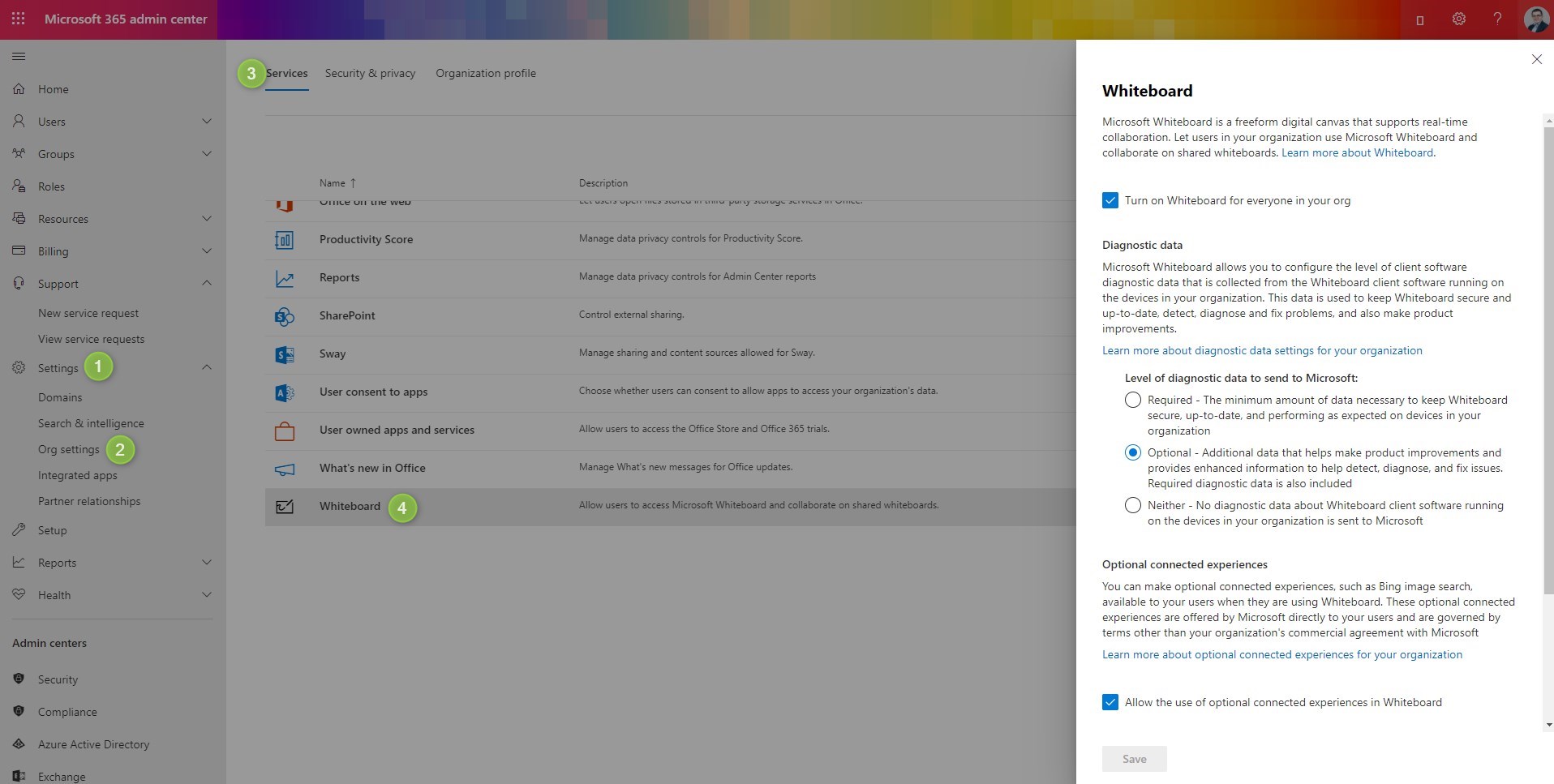This is a composite image, comprising two overlapping screenshots related to Microsoft 365. The primary screenshot appears to be from the Microsoft 365 Admin Center, featuring a minimalistic white interface with a top navigation bar adorned with a thin, rainbow-colored strip in shades of pink, blue, burgundy, green, yellow, gold, and red. The strip includes icons such as a white cogwheel (likely for settings), a white question mark (possibly for help), and a small circular profile picture, which is too tiny to discern any specific details.

Below the profile picture is a white pop-up window with predominantly black text, providing information about the Microsoft Whiteboard feature. It includes a blue checked box captioned "Turn on Whiteboard for everyone in your organization." Additionally, there is a section labeled "Diagnostic data," accompanied by a blue circle and further black text.

In the background, the secondary image displays a submenu on a white backdrop showcasing various administrative settings. Visible options include "Home," "Users," "Groups," "Accounts," "Billing," "Support," among others. This section features organized, streamlined services, represented by green circles with white text, indicating selectable menus. The secondary image further elaborates on available settings and options within the Microsoft 365 Admin Center. The overall visual captures the clean and user-friendly design of Microsoft's administrative interface, emphasizing accessibility and functionality.